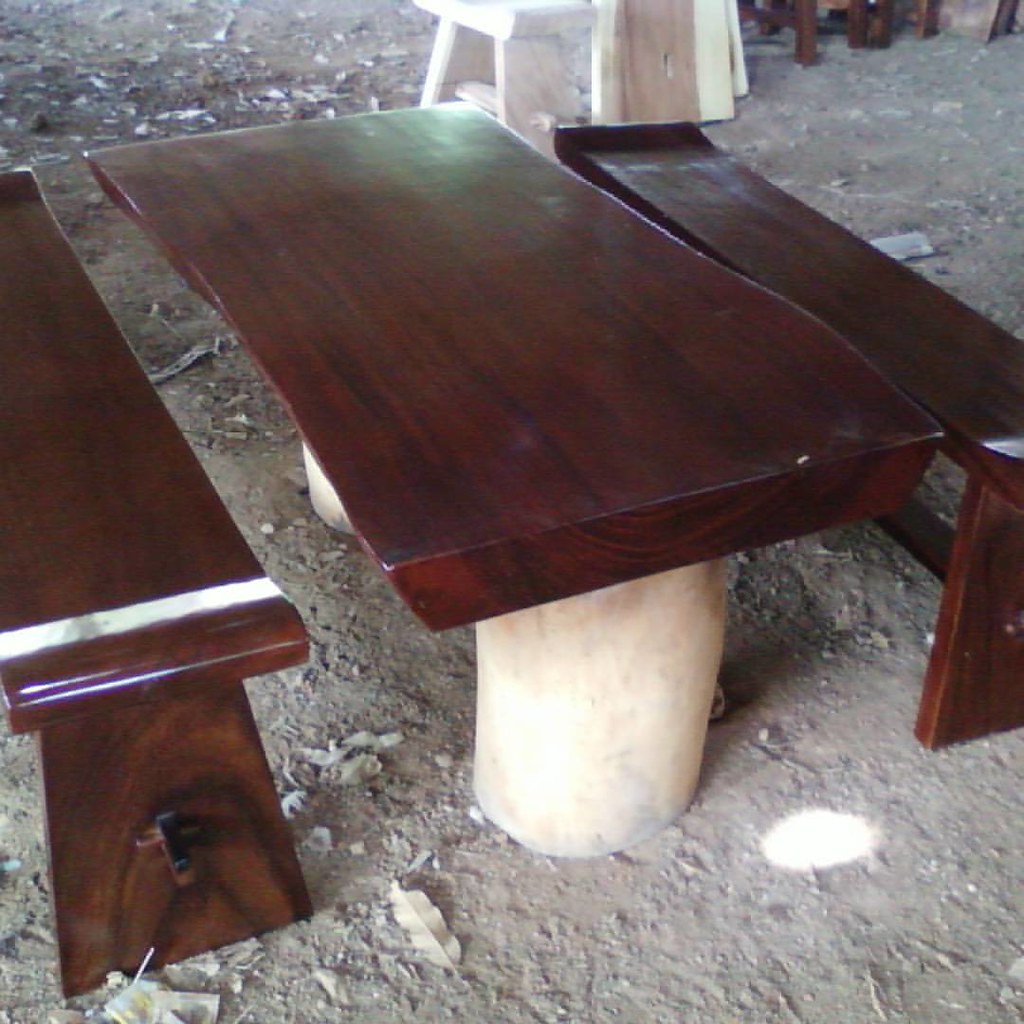This image depicts an outdoor eating area featuring a large red oak table on two beige, round concrete piers. The table has a middle section that's wider than its matching benches, with a distinctive thick and uneven edge that almost appears broken. The tabletop showcases rich wood grains similar to those on the benches, which may be stained a dark cherry color. One bench has a white stripe running across its top, while the other seems to have a similar stripe, partially visible. The area around the furniture is a dirt patch with scattered leaves, twigs, and no grass. Various unfurnished wooden items are visible in the background, hinting at additional seating or tables. The scene might be under some sort of overhead cover.